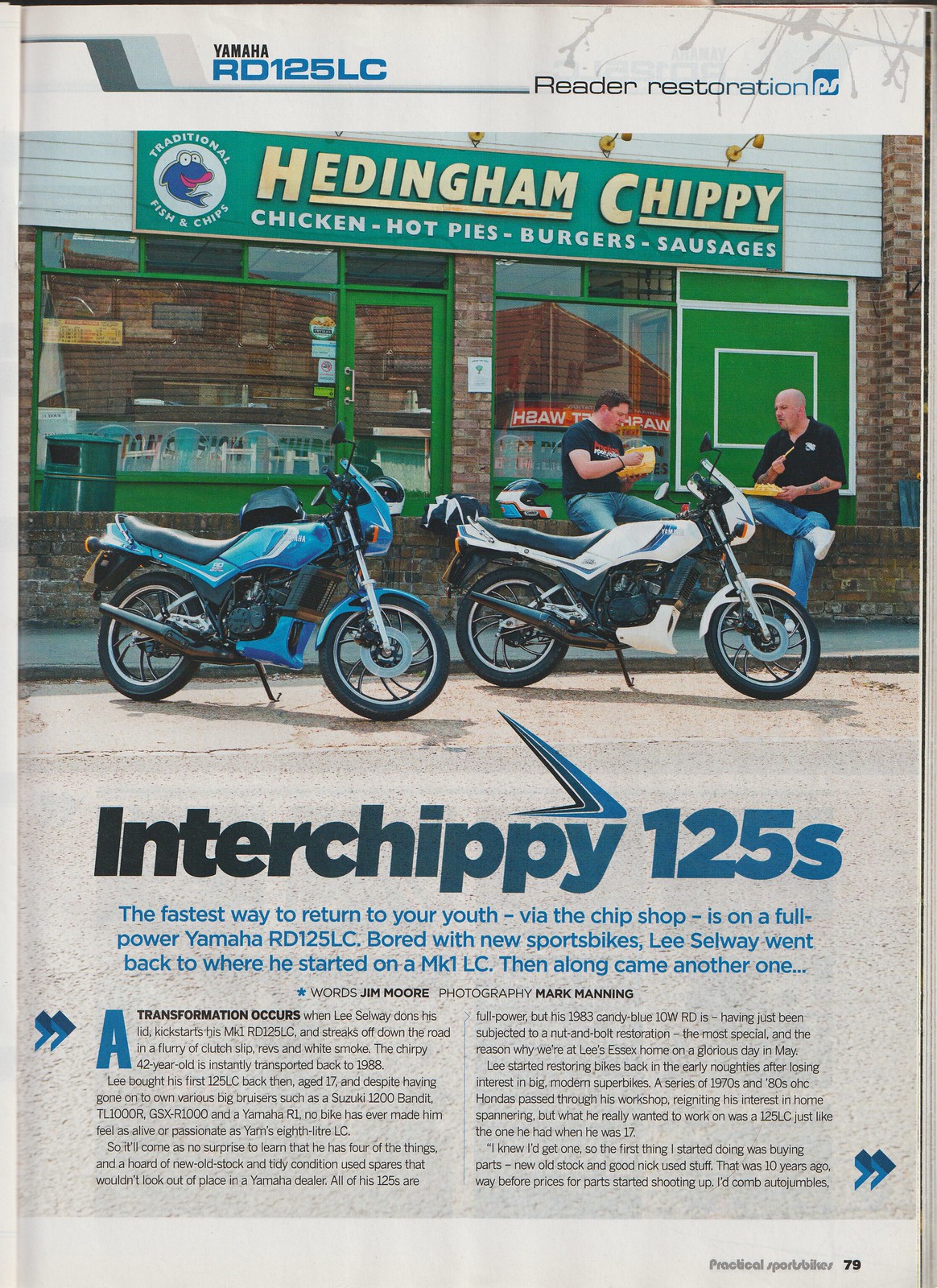This is a color photograph of a restored magazine article titled "Yamaha RD 125 LC Reader Restoration." At the top of the page, the text announces "Interchippy 125 S.” The tagline reads, "The fastest way to return to your youth via the chip shop is on a full power Yamaha RD 125 LC. Bored with new sports bikes, Lee Selway went back to where he started on an MK1 LC. Then along came another one..."

Below the text is an image of a green and brick restaurant with large glass windows and the name "Headingham Chippy" prominently displayed in yellow letters. The restaurant advertises Chicken, Hot Pies, Burgers, Sausages, and Traditional Fish and Chips. 

In front of the restaurant, two motorcycles are parked with their kickstands down: one is blue, and the other is black and white. To the right of the glass window and door, two men are seated on the brick sidewalk, each eating from yellow takeout containers. Both men wear blue jeans, white tennis shoes, and short-sleeve black t-shirts; the man on the left has short dark hair, while the man on the right is bald. 

Beneath this photograph, the page transitions into two columns of small, indecipherable black text, indicating further content likely reviewing the motorcycles and their nostalgic appeal. The magazine appears to be open to page 79, hinting it’s part of a larger collection of similar content.